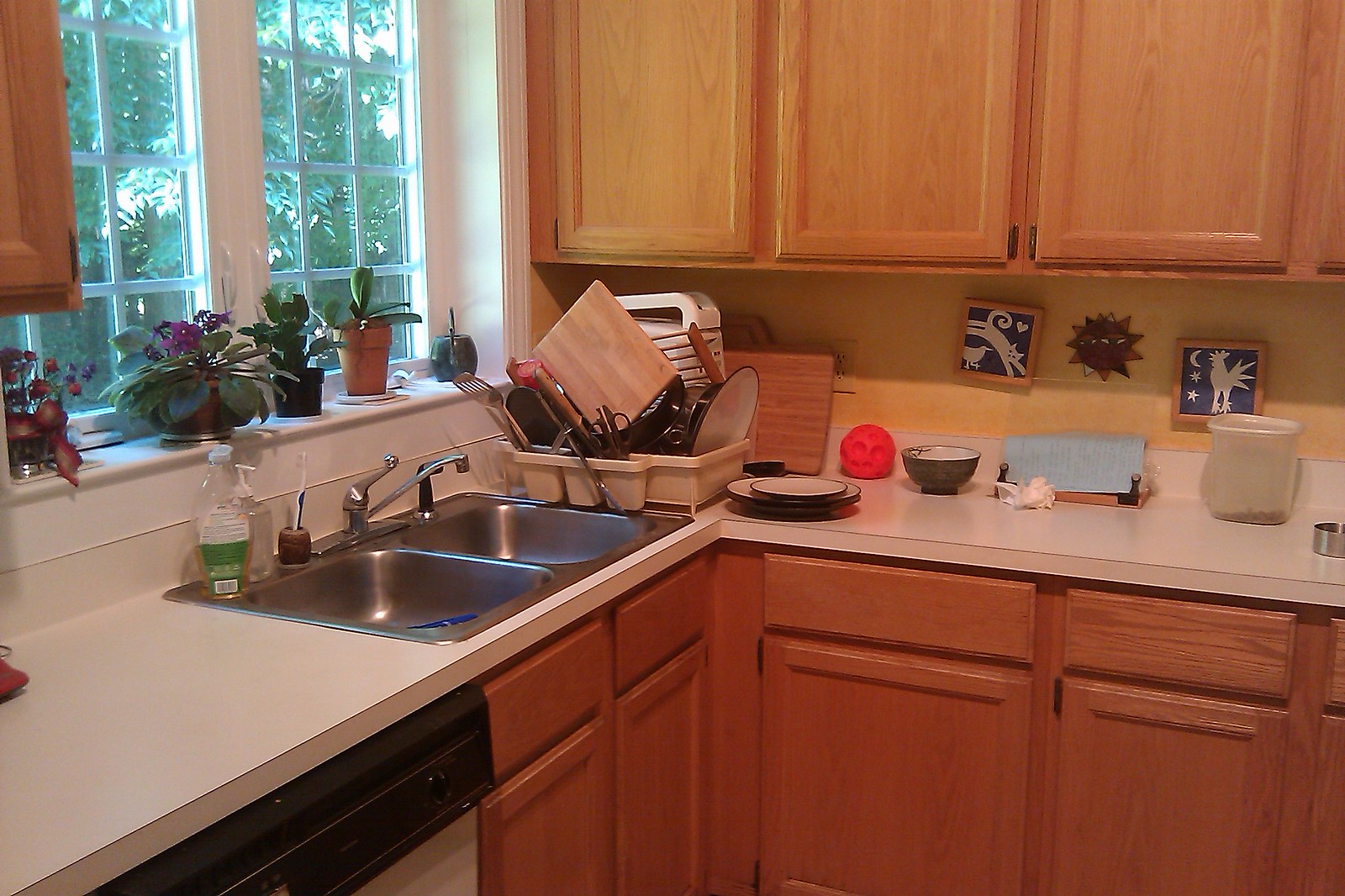A clean and well-organized kitchen is depicted in this image. The kitchen features light brown cabinetry, with three upper cabinets extending from the upper right corner to more than halfway to the upper left corner of the image. Beneath these cabinets, a countertop is visible, holding a dish drainer filled with various dishes and silverware. Next to the dish drainer, there is a small stack of three plates, a bowl, and a paper towel holder. The wall behind the countertop is adorned with a couple of small pictures featuring celestial-themed images.

To the right of the countertop, the layout shifts vertically, revealing a double kitchen sink made of silver metal. Above the sink is a window, and the windowsill is decorated with four mini potted plants, including two flowering plants with purple and red blooms. In the bottom left corner of the image, the edge of a dishwasher is just visible. Completing the scene, there are two additional lower cabinets next to the dishwasher, contributing to the kitchen's neat and functional appearance.